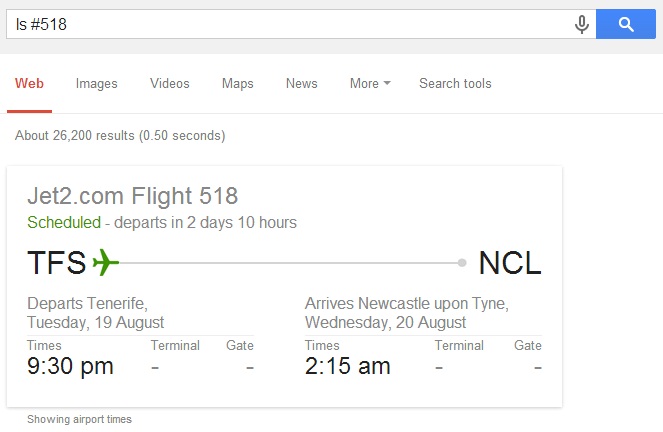A screenshot captured on an Android or Google phone, evident from the angular design of the search bar typically not found on Apple devices, shows a Google search for "IS 518." The search results include an automated pop-up providing detailed flight information for Jet2.com flight 518. This flight is scheduled to depart from Tenerife (TFS) and arrive in Newcastle upon Tyne (NCL) in two days and ten hours. Currently, terminal and gate information are not available, suggesting they will be updated as the departure time approaches. The status indicates the flight has not yet departed, shown by a green airplane icon positioned at the TFS end of a grey progress line, signifying the plane's current location.